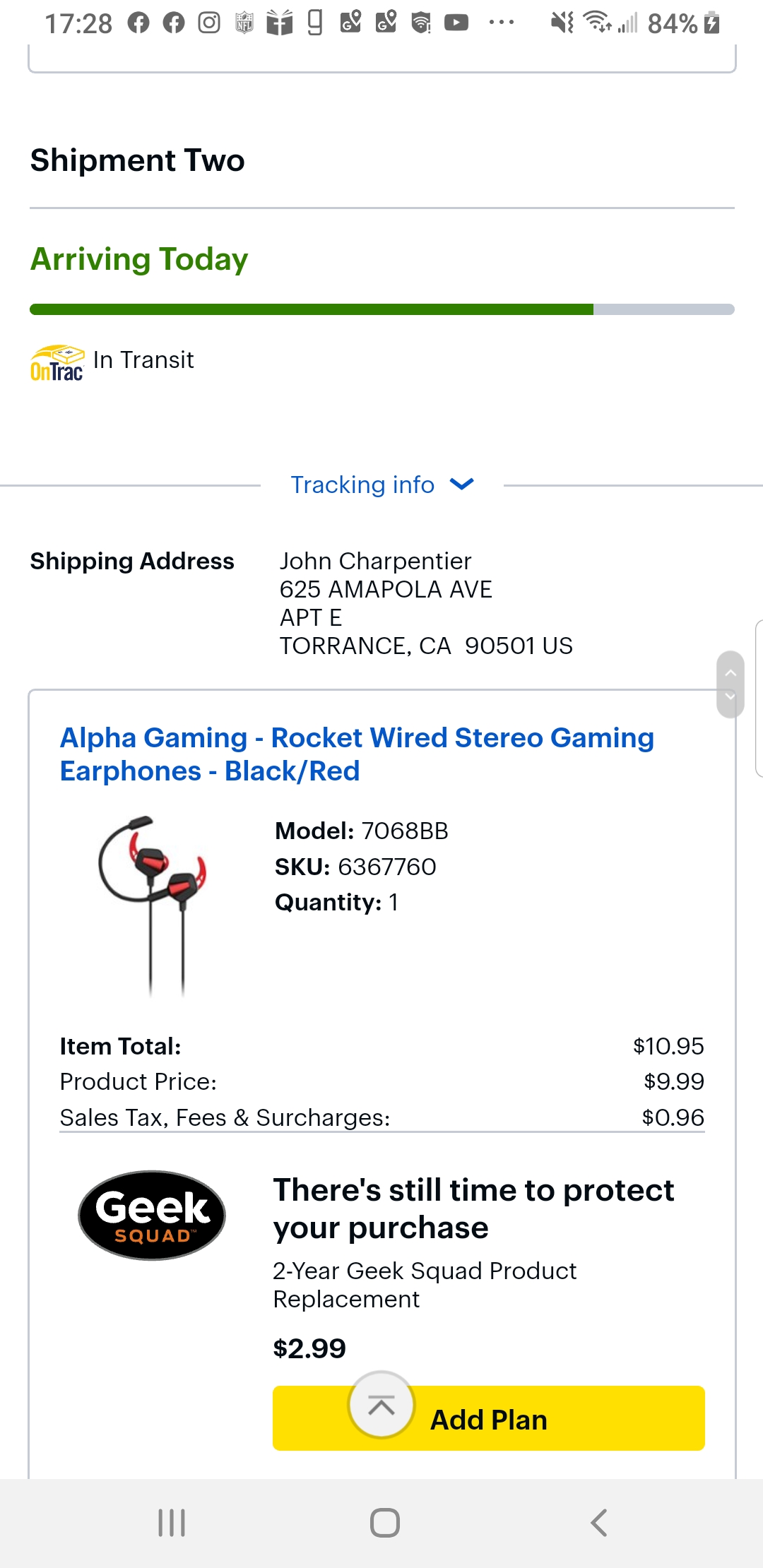The image displays the Best Buy website on a mobile phone screen. At the top, the status bar shows the time as 17:28, along with various icons including Facebook, Instagram, and the battery percentage indicator. Below the status bar, the webpage section begins, containing shipment details.

A black text header reads "Shipment to" with "arriving today" highlighted in green, accompanied by a nearly full green progress bar. Below this, status indicators show "In transit" and "On track" to the left. The "Tracking info" link is prominently displayed in blue.

The shipping address is clearly listed:
- John Carpentier
- 625 Amapola Avenue, Apartment E
- Torrance, CA 90501 US

Within a gray-bordered box, the details of the ordered item are presented. The product is "Alpha Gaming Rocket Wired Stereo Gaming Earphones" in black and red, with a photo showing the earphones and microphone. Key product specifications are:
- Model: 7068BB
- SKU: 6367760
- Quantity: 1
- Item total: $10.95
  - Product price: $9.99
  - Sales tax, fees, and surcharges: $0.96

The page also features a Geek Squad promotional message urging the customer to protect the purchase. It offers a "two-year Geek Squad product replacement" plan for $10.99, with a yellow "Add plan" button readily accessible.